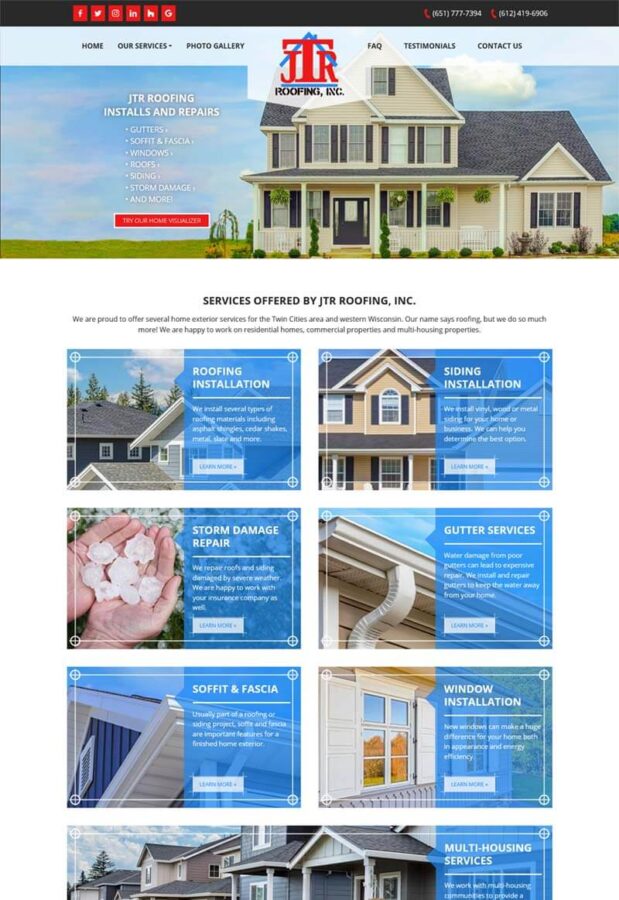A highly detailed and polished caption for the image could be:

"The website appears to belong to a contractor, prominently showcasing their services. At the top, there is a panoramic image of a two-story beige house with a gray composition roof, set against a blue sky backdrop. On the left side of the image, 'JTR Roofing Installs and Repairs' is displayed in crisp white lettering. Beneath this header, the webpage is divided into two columns, each featuring three pictures. The first column displays images related to 'Roofing Installation,' 'Storm Damage Repair,' and 'Soffit and Fascia.' The second column highlights services such as 'Siding Installation,' 'Gutter Services,' and 'Window Installation.' Each picture is accompanied by a brief description of the corresponding service, providing a clear visual and textual representation of the contractor's offerings."